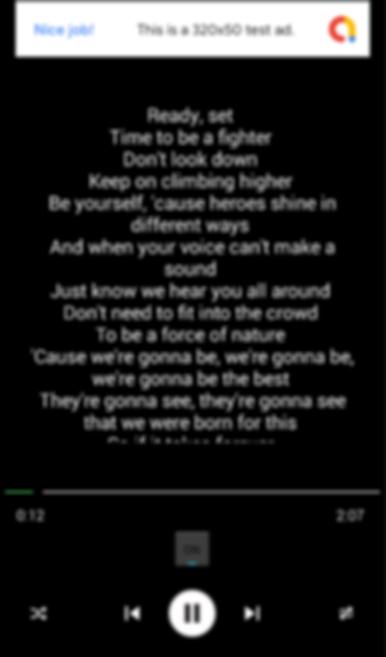This image is a screenshot featuring text formatted in a visually poetic style, with words centered and expanding outwards in different stanzas. At the top, the search bar is faint and slightly blurred, displaying a partial and unreadable text that seems to suggest "nice job, this is a 5, 20."

The primary text in the image follows, reading:

"Ready, set,
time to be a fighter,
don't look down,
keep on climbing higher.

Be yourself,
'cause heroes shine in different ways.
And when your voice can't make a sound,
just know we hear you all around.

Don't need to fit into the crowd
to be a force of nature,
'cause we're gonna be,
we're gonna be,
we're gonna be the best.
They're gonna see,
they're gonna see,
that we were born for this."

Below these lines, there seems to be another part of the text that is not visible in the screenshot. At the bottom of the image, there is a button, suggesting the possibility that this text might be auditory in nature, indicated by its label as a "start" button. This button implies that there may be an option to listen to the text rather than read it.